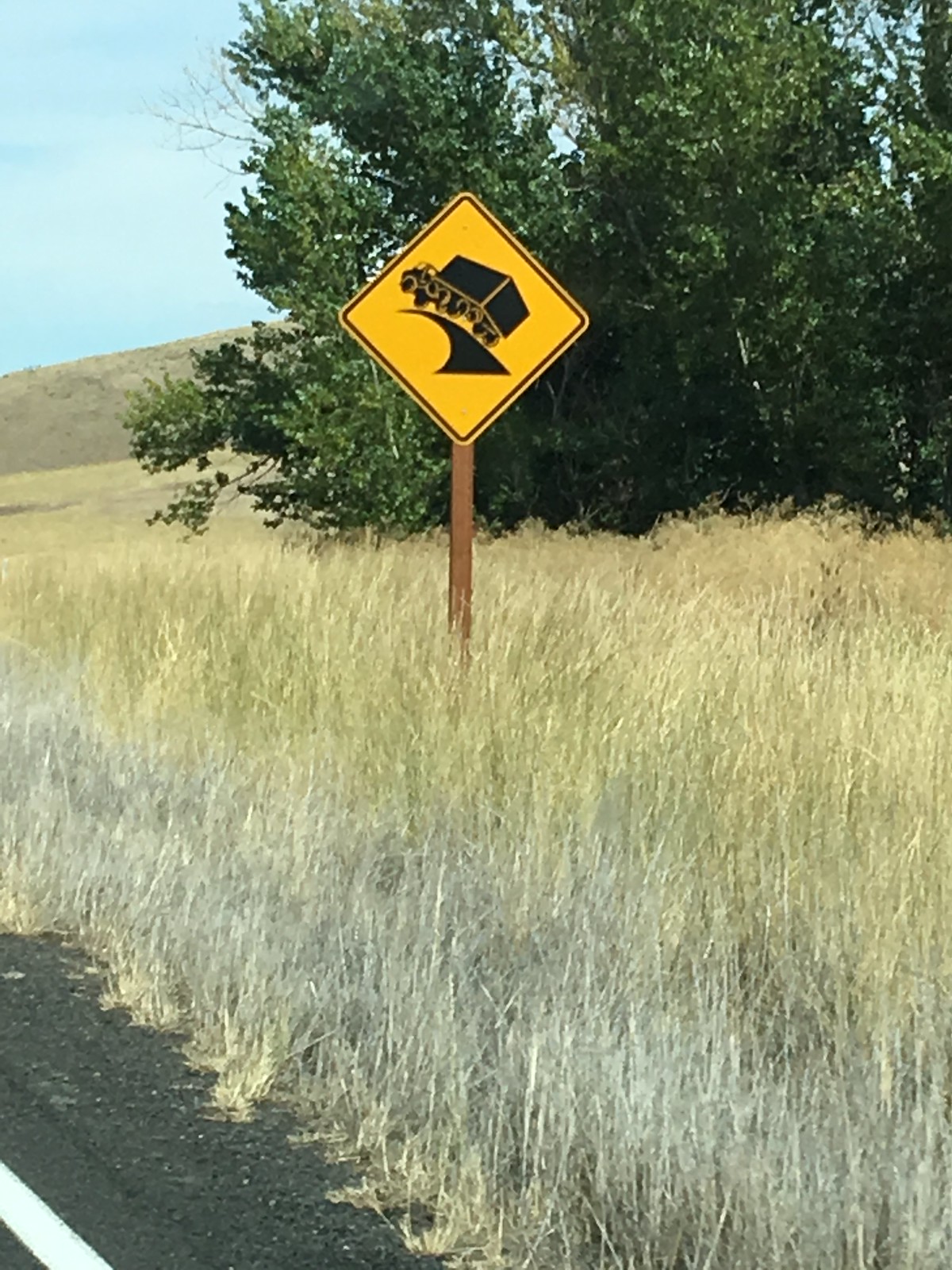This grainy photograph, taken from the roadside, captures a scene dominated by a tall, wild, and slightly dead grass field stretching into the distance. In the bottom left corner, there's a touch of asphalt featuring a thick white line marking the side of the road. A prominent yellow diamond-shaped road sign with a black border commands attention near the road. The sign, displaying a black image of a truck leaning as it navigates a curve, warns about the tipping hazard ahead. Close to the road, a few green trees tower up to the top of the image, adding depth to the scene. In the distance, gently rolling green hills rise toward the right, set against a blue sky streaked with faint, wispy clouds.